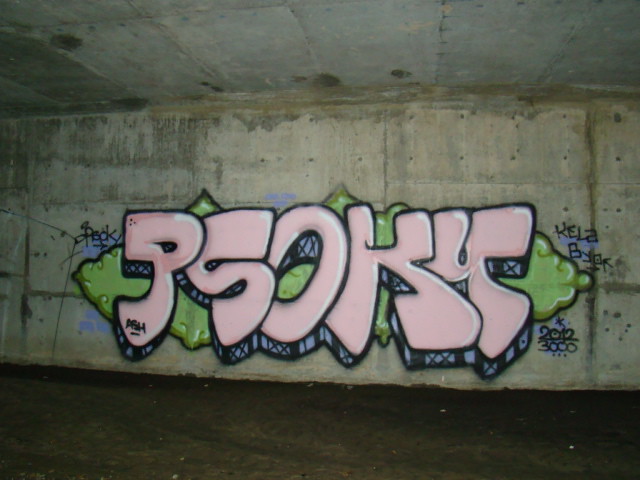The color photograph captures an outdoor scene that appears to be situated either within a tunnel or beneath a bridge, characterized by extensive concrete structures. The main focus is a large concrete wall, complemented by a concrete ceiling and floor, all of which exhibit a rough texture. The concrete floor is notably darker and possibly wet, adding to the overall ambiance of the location.

Dominating the concrete wall is a piece of stylized graffiti featuring the letters "P-S-O-K-Y" rendered in a prominent pale pink and lime green color scheme. The background of the graffiti includes lime green clouds and additional splashes of light blue and black, enhancing the visual complexity. Surrounding the primary graffiti are various other writings and markings. On the left side, there are words that could be "P-E-C-K-Y" or "B-E-C-K-Y," though these are slightly distorted and distant in the image. On the right side, the text "K-E-L-A-B-Y-O" is visible, followed by the letters "K" and the numbers "2012" and "3000" directly below.

The setting is dimly lit, suggesting the use of a camera flash to illuminate the scene, which reveals spots on the walls indicative of water or mold damage. The photograph provides a detailed glimpse into an urban, likely neglected, concrete environment adorned with vibrant street art.